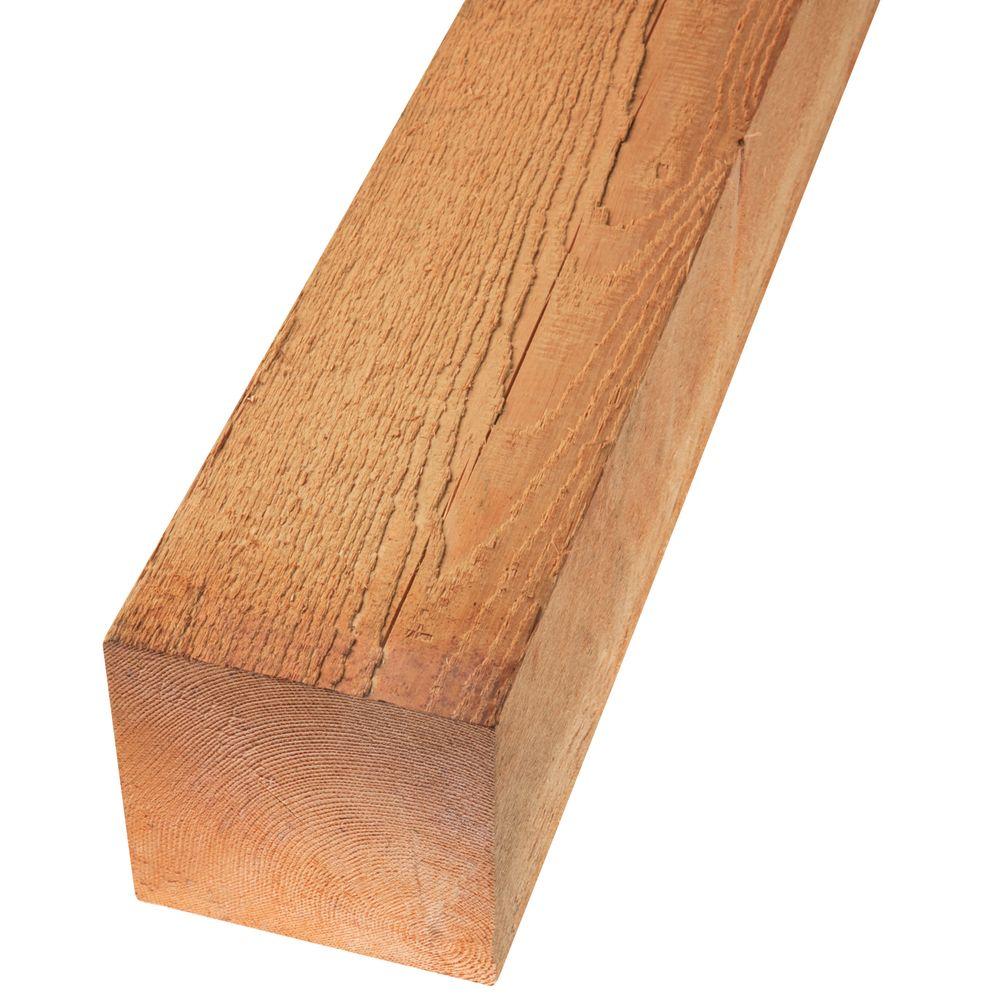The image features a vertically oriented piece of 4x4 lumber against a white background. The wood displays a variety of brown tones, from light brown on its top surface to darker shades with a reddish tint on its sides. The top, which is cut and sanded smooth, showcases detailed grain textures, ripples, and small cracks. This surface is worn and streaked, highlighting the natural tree rings and intricate patterns in the wood. The front edge of the lumber is also visible, revealing additional tree lines and a slightly golden finish that suggests a possibly treated or stained surface. The piece extends from the top to the bottom of the image, giving a partial view that emphasizes the lower section.